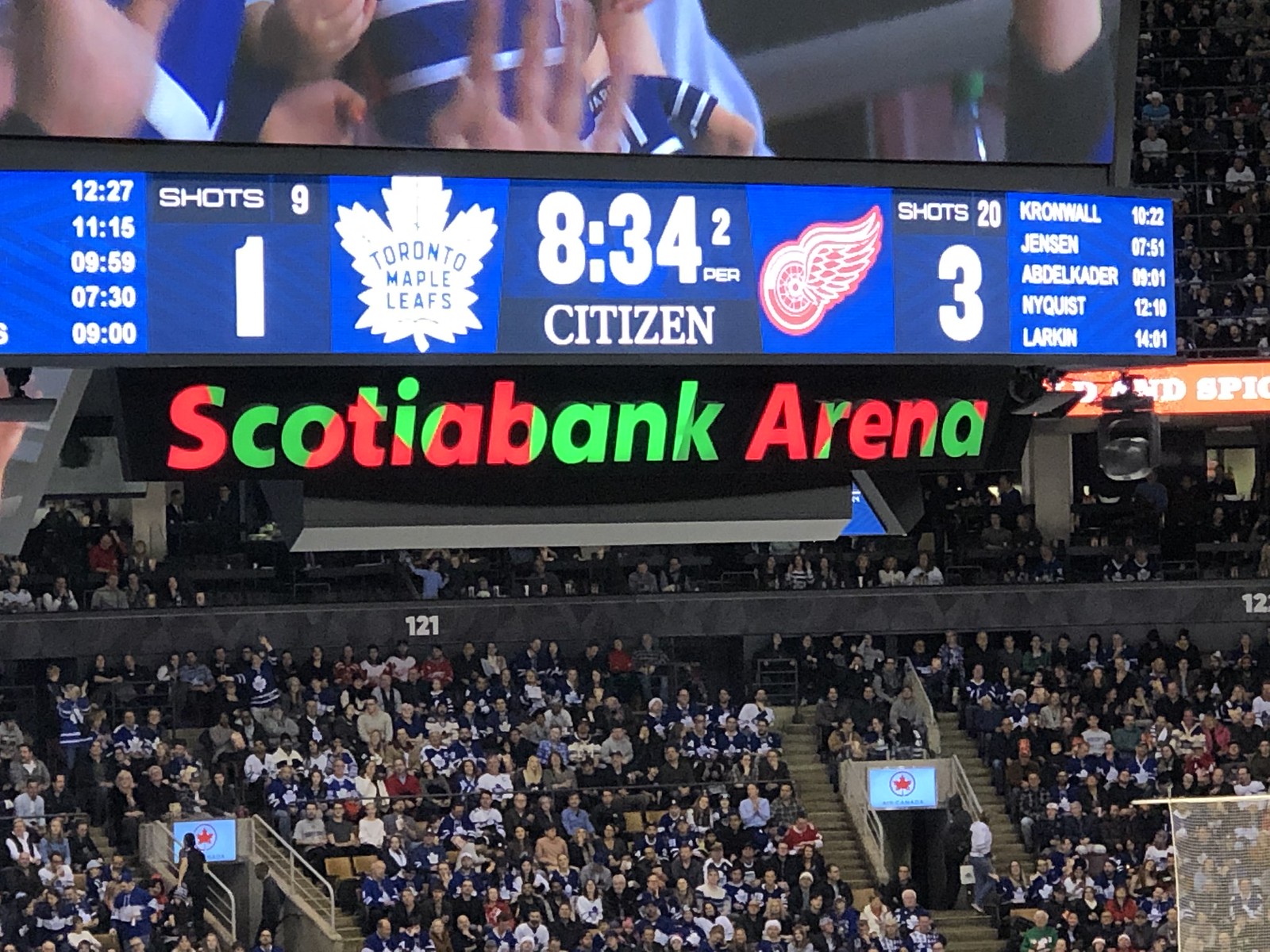This photograph captures a bustling indoor scene at Scotiabank Arena in Toronto, Canada, during an intense hockey game. The audience fills the seats almost completely, showcasing a sea of excited spectators. In the foreground, rows of seats and staircases can be seen, with people sitting eagerly and watching the game. Central to the image is a large scoreboard and a giant television screen displaying crucial game details. The Toronto Maple Leafs are trailing the Flyers with a score of 1 to 3, indicated alongside their respective shot counts—9 for the Maple Leafs and 29 for the Flyers. The time displayed shows 8 minutes and 34 seconds remaining in the second period. Players' names, including Cromwell, Jensen, Addo, Cole, and Larkin, are listed on the board. The image is awash with colors such as blue, white, dark blue, black, gray, orange, and green, contributing to the vibrant atmosphere. The clearly visible Scotiabank Arena sign affirms the location within this lively indoor setting.